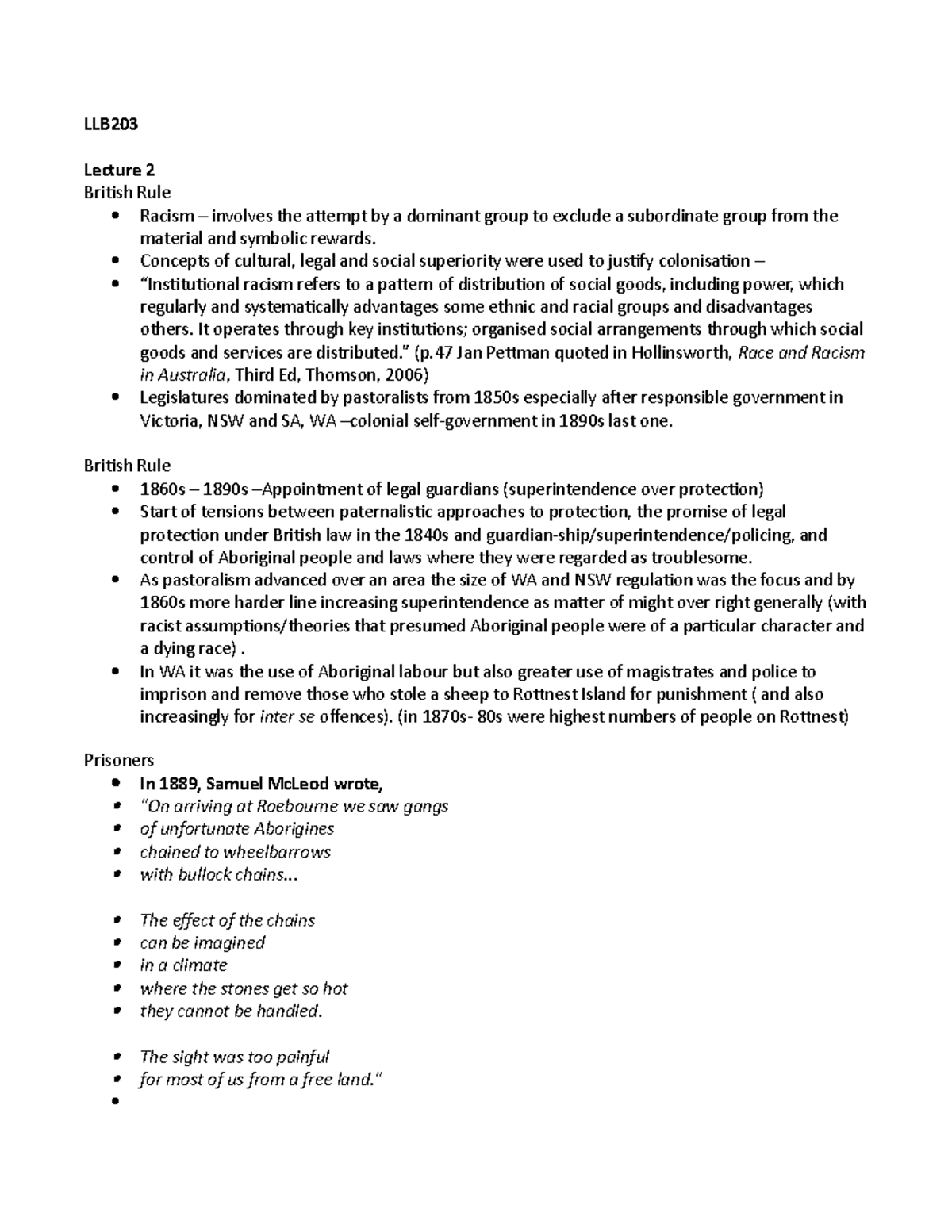**Caption:**

The image features an entirely white background with black font, formatted with bullet points. The text details topics related to British Rule, as part of Lecture 2 for LLB203:

- **Racism**: Defined as the attempt by a dominant group to exclude a subordinated group from material and symbolic rewards.
- **Colonization Justification**: Concepts of cultural, legal, and social superiority were used to justify colonization.
- **Institutional Racism**: Described as a pattern of the distribution of social goods and power that systematically advantages certain ethnic and racial groups while disadvantaging others. This form of racism operates through key institutions and organized social arrangements responsible for the distribution of social goods and services. Quoted from Jan Peterman in Hollingsworth's "Race and Racism in Australia," 3rd edition, Thomas, 2006, page 47.
- **Legislative Dominance**: Pastoralists dominated the legislature from the 1850s, especially after responsible government was established in Victoria, New South Wales, South Australia, and Western Australia—leading to colonial self-government in the 1980s.
- **British Rule Timeline**: 1860 to 1990s.

Each bullet point is succinctly detailed, providing a comprehensive overview of key topics discussed in the lecture.